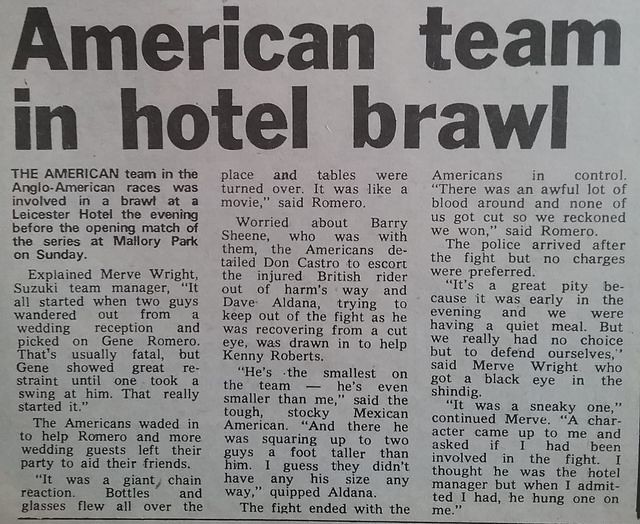This image features a vintage newspaper clipping with a bluish-gray background, giving it an aged appearance. The article is titled, "American Team in Hotel Brawl," printed in large, bold black letters at the top left. The content is organized into three columns of black text. The upper left-hand column includes the bolded introductory paragraph, which reads, "The American team in the Anglo-American races was involved in a brawl at a Leicester hotel the evening before the opening match of the series at Mallory Park on Sunday." Additional details are mentioned in the main column, explaining the incident: "Suzuki team manager Merv Wright described how the brawl commenced when two individuals wandered from a wedding reception and targeted Gene Romero. Although Romero initially showed restraint, the situation escalated when one of the individuals took a swing at him, prompting the American team to intervene." The clipping appears to have been photographed up close or cut out from its original source, and no date or author is visible. In the lower right-hand corner, there is a noticeable thick black line fragment. Overall, the image captures a crucial moment reported in this historical newspaper article.